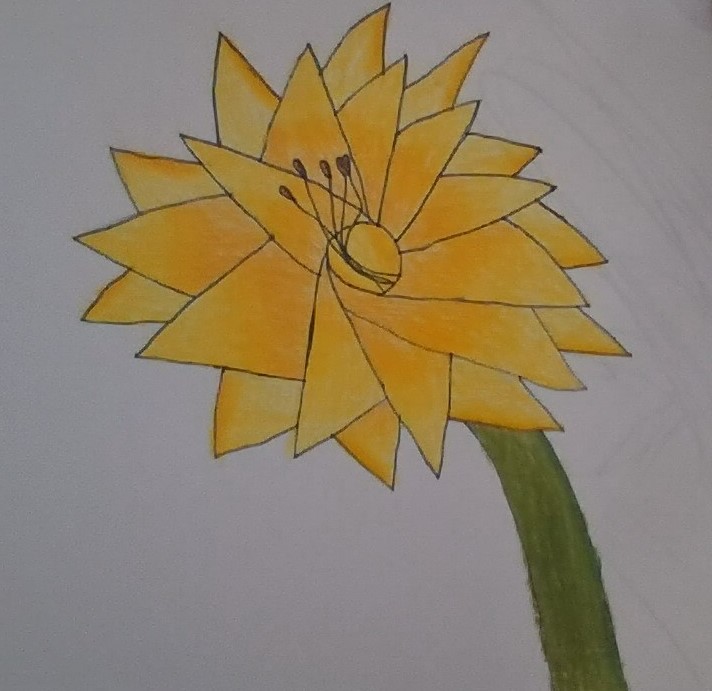This image features a vivid illustration, possibly rendered with colored pencils, set against a stark white background suggesting it was created on white paper. The artwork depicts a stylized flower with an emphasis on modern, abstract design elements. Dominating the composition, the flower exhibits bright yellow petals and a green stem. Although only a small portion of the stem is visible, the focus is clearly on the flower itself. The center of the flower is a circular core, filled with elements that resemble seeds. Surrounding the core is a series of asymmetric triangles that form the petals, giving the flower a unique, geometric appearance. This vibrant and youthful illustration, with its simple yet sophisticated design, exudes a playful charm, hinting at the creative expression of a student or someone embracing a childlike perspective.